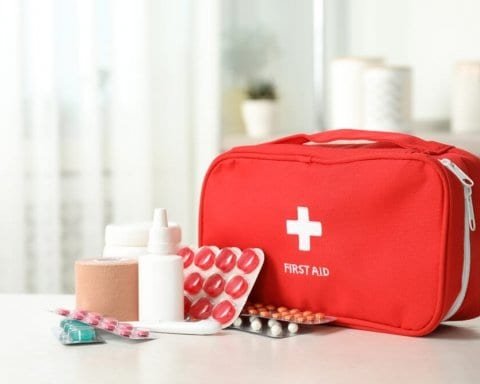This detailed photograph depicts a red first aid kit prominently placed on a white countertop. The red canvas bag features a white cross at its center and bold, white all-caps letters spelling "FIRST AID" just below the cross. The bag, equipped with white zippers and a red handle, is surrounded by an assortment of medical supplies typically found within such a kit. 

In front of the bag lies a mix of items: a small, white plastic bottle, packets with various pills—some green, some orange, and others red, along with a packet containing medicine in a silver foil. Among these supplies are also some brown gauze tape and circular red pill packets standing upright. 

The setting appears to be a room with a blurred but dominantly white background. On the left side, vertical sheer white curtains are visible, partially covering a window. Beside the curtains, a white vase with a green plant peeks out, and a nearby shelf holds what looks like paper towels. Additionally, a silver metal pole vertically bisects the scene, accompanied by three more white pots to its right.